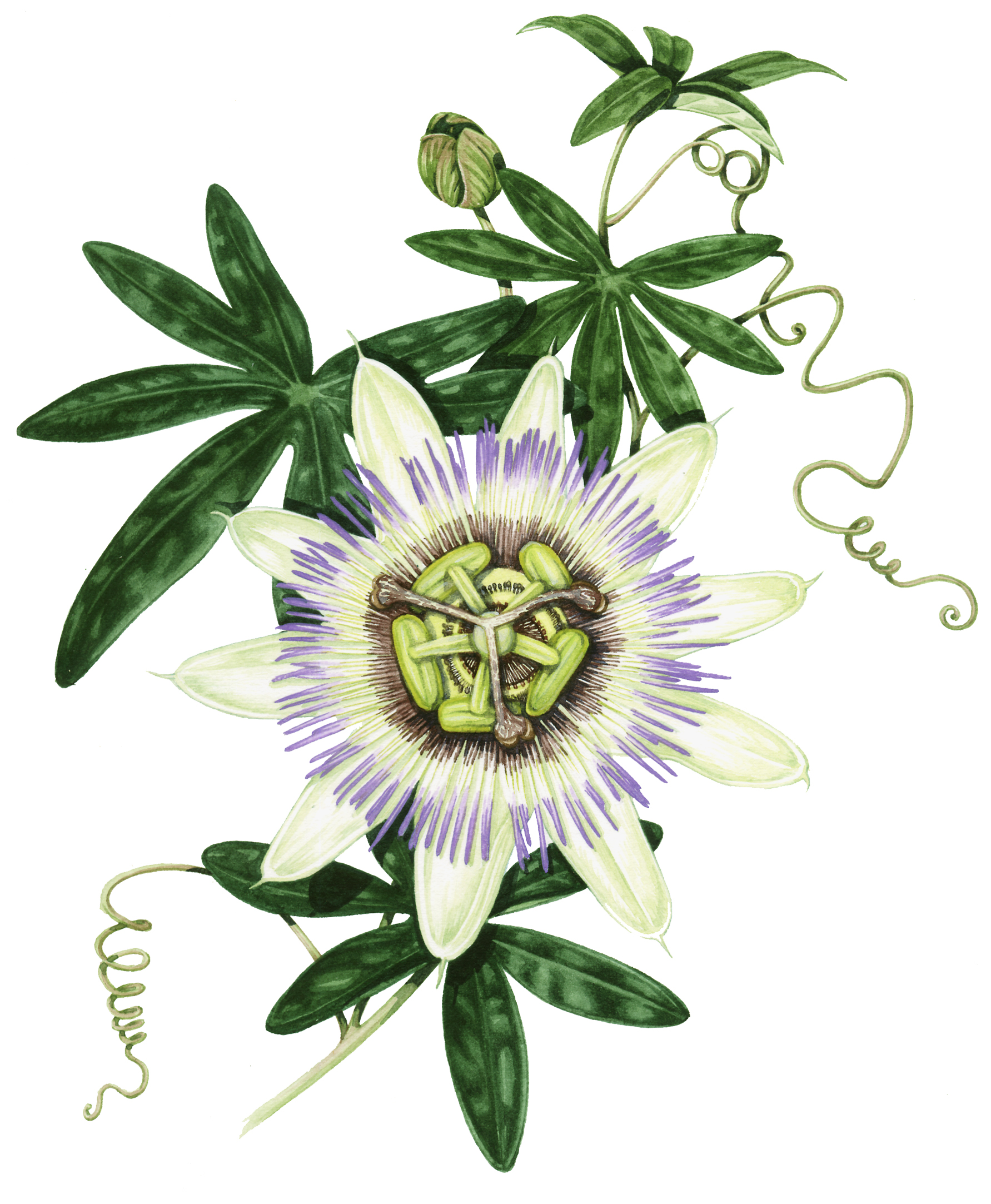This is a detailed, hand-drawn or painted image of a flower on a white background. The focal point is a white flower with ten delicate, stringy petals. The base of the petals is dark brown, transitioning to white and then purple at the tips. Surrounding the center of the flower in a full 360-degree arrangement, these petals encircle a central region that features green, oval-shaped structures reminiscent of kidney beans. Additionally, there appears to be a three-pronged nucleus at the heart of the flower.

Branching off the light green stem, which ascends from the bottom of the image, are curly vines that form little spirals. The stem supports various green leaves that are elongated and oval-shaped, including a set below the flower, each with six to seven points. These leaves have a star-like appearance and add a dynamic touch. At the top of the image, there is another flower bud that has yet to bloom. The composition as a whole gives a sense of meticulous detail and vibrant color contrast between the flower and its surroundings. There is no text present in the image.